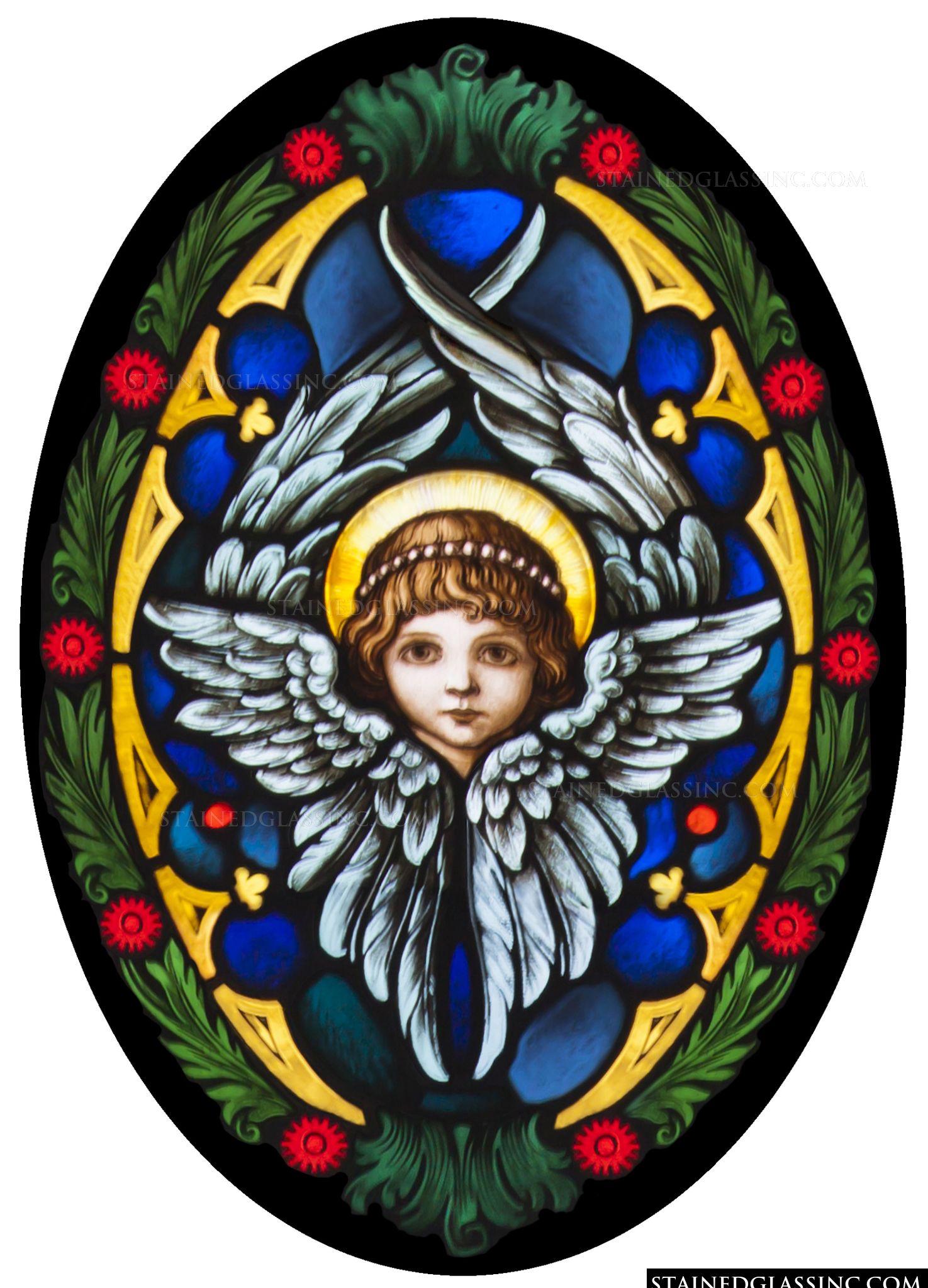This image features a detailed stained glass mosaic set against a plain white background, with "stainedglass.com" watermark in the lower right corner. The piece is oval-shaped with a prominent black outer border. Just inside the black border, a wreath-like design of green leaves interspersed with red flowers encircles the artwork. Moving inward, there is a ring of gold elements featuring four fleur-de-lis. Next comes a blue ring of stained glass tiles, followed by yellow triangular designs. 

At the center of the piece is the focal point: an angelic figure with a face framed by auburn hair and adorned with a crown-like headband of pearls. A vivid golden halo radiates behind the head of the angel, while its serene face is surrounded by white angel wings that extend from the neck upwards. The colors across the design—blue, gold, and green—are sharp, bright, and vividly showcased, suggesting that this mosaic would be especially brilliant when illuminated by sunlight.